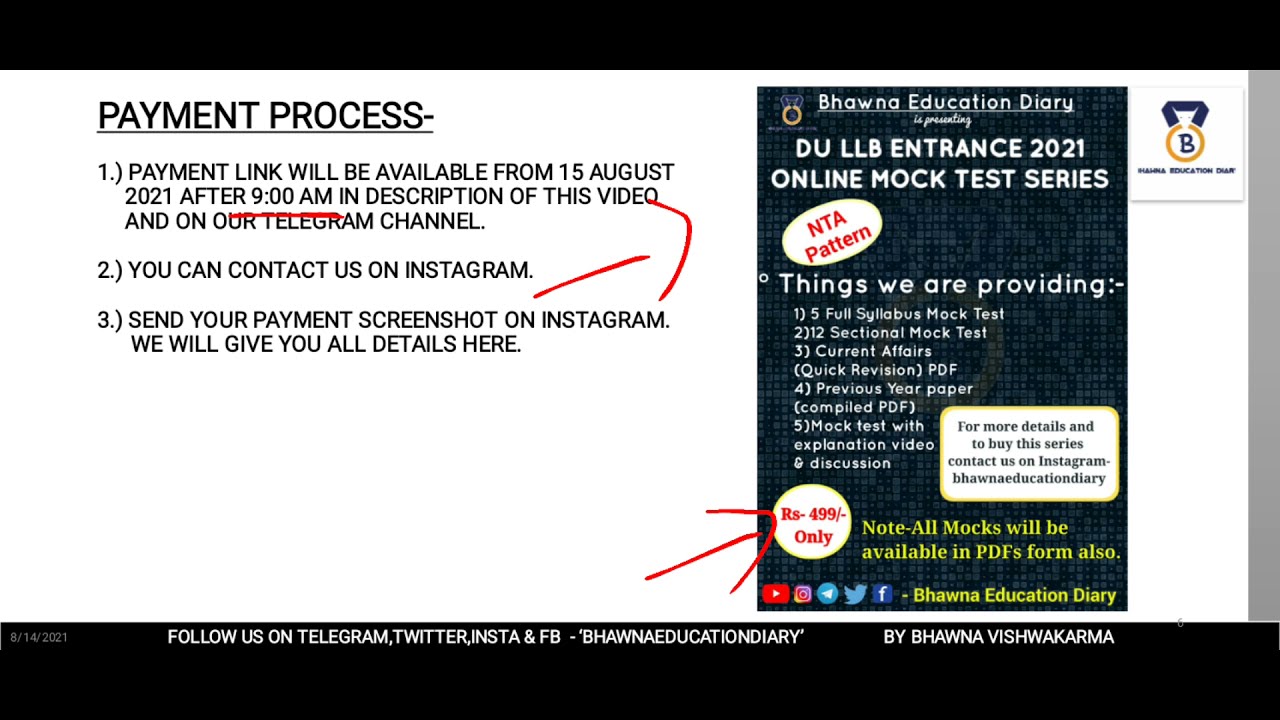The image is a computer-generated advertisement primarily featuring a "Payment Process" segment on a white background with black borders at the top and bottom. The top black bar is long, while the bottom one is slightly larger. In the bottom bar, white font instructs viewers to follow "Bahuana Education Diary" on Telegram, Twitter, Instagram, and Facebook. 

On the left side of the image, in black lettering, it details the payment process. It outlines:
1. "Payment link will be available from 15 August 2021 after 9 a.m. in the description of this video and on our Telegram channel." The text "9 a.m." is underlined in red, and "Telegram" is crossed out in red.
2. "You can contact us on Instagram."
3. "Send your payment screenshot on Instagram. We will give you all details here."

A red arrow is drawn, pointing to a blue vertical rectangle on the right side, advertising the "DULB Entrance 2021 Online Mock Test Series" by Bahuana Education Diary. This ad lists:

1. 5 full syllabus mock tests
2. 12 sectional mock tests
3. Current affairs quick revision PDF
4. Previous year papers
5. Mock tests with explanation videos and discussions

For more details and to purchase the series, viewers are directed to contact "Bahuana Education Diary" on Instagram. Additionally, a small white box notes that all mocks will be available in PDF form. In the upper-right corner of the image, there is an icon of a medal with the text "Be On." The image encompasses the educational resources provided for the DULB entrance exam and the associated payment instructions, with comprehensive contact information and social media prompts.